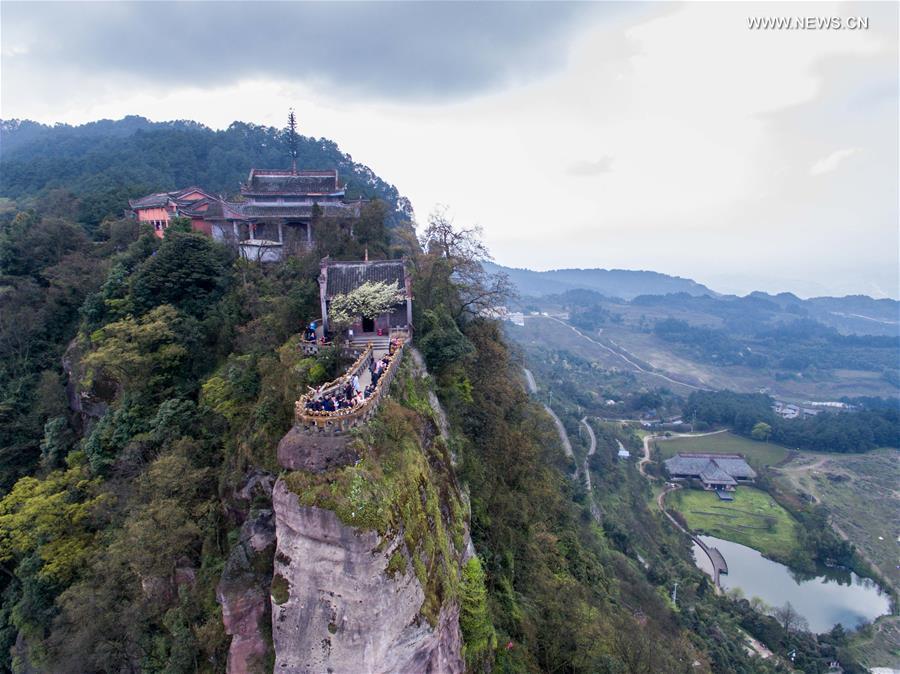In this outdoor aerial shot, a large gathering of people stands atop a cliffside, encircled by a stone banner, peering out at the expansive landscape. Behind them, a pathway leads to several buildings: a red one with a black roof on the left, and two slightly larger gray-blue structures with darker roofs. The cliff and surrounding mountain range are densely covered in various shades of green foliage. To the right, the valley reveals a serene lake and a road that winds past another lighter-colored building with a gray roof, continuing toward a hillside dotted with smaller structures. The sky is notably overcast, filled with dark gray clouds, enhancing the dramatic and moody atmosphere of this detailed outdoor scene. The setting is lush and vibrant despite the darker sky, with unique hills, grasses, and bodies of water contributing to the picturesque view.